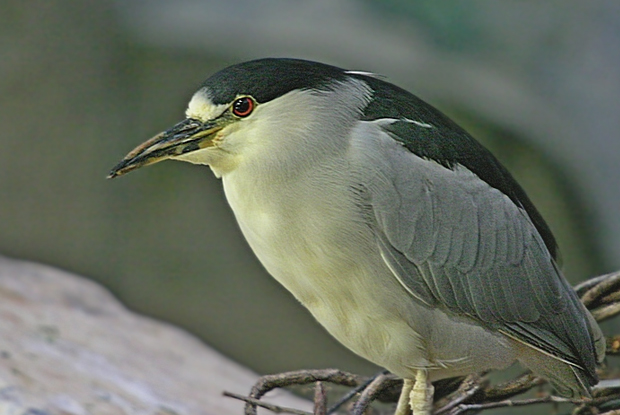This image features a bird, facing to the left, with a distinctive red coloration around the bottom edge of its eye. The bird's wings are white, while its body displays a mix of black on the top part of its head and back, complemented by some greenish hues. The beak is notably long, exhibiting a blend of yellow, green, and a hint of orange. The bird appears to be perched on a branch or possibly a nest, though the exact footing is obscured and indistinct. The bird's feet are not visible. The background is completely out of focus, making it hard to discern specific details, though it vaguely maintains a color palette similar to the bird’s greenish-gray tones. In the bottom left corner of the image, there seems to be a rock or a rock surface associated with the area where the bird is standing.